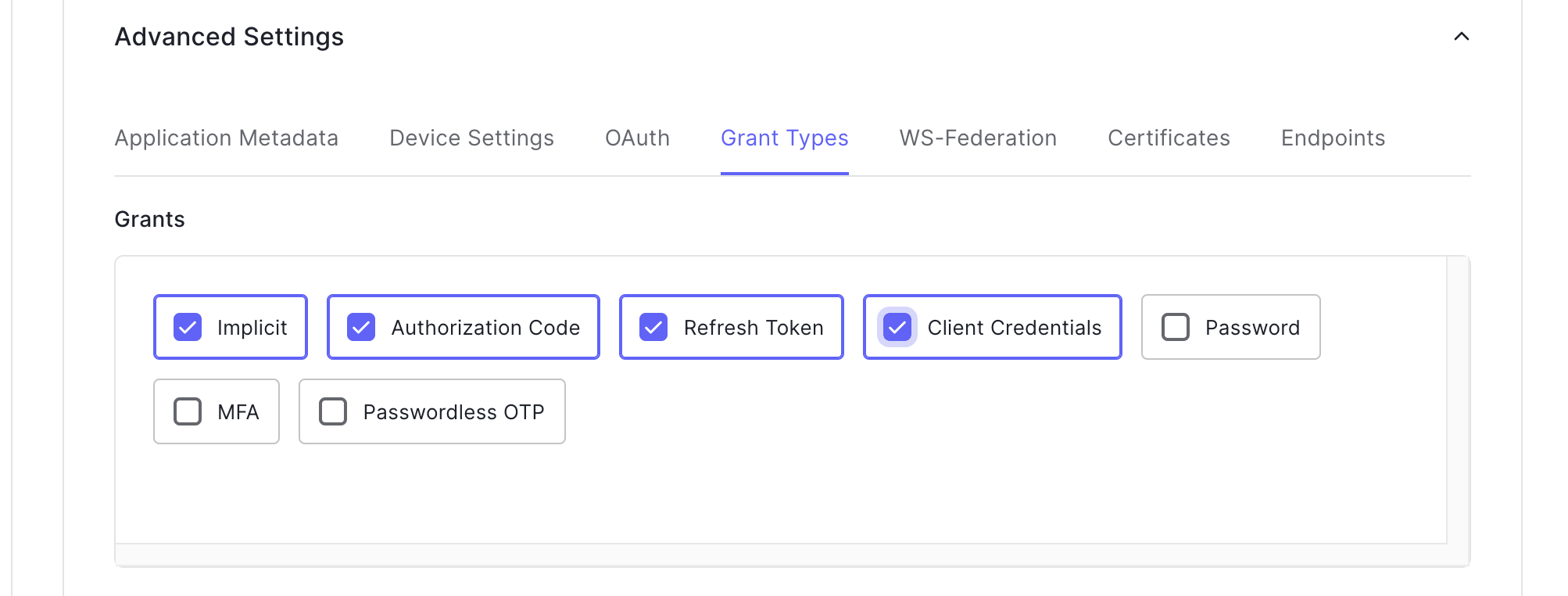The image depicts a settings page with a white background titled "Advanced Settings" at the top left. Below this title, a series of tabs are arranged horizontally: "Application Metadata," "Device Settings," "OAuth," "Grant Types" (highlighted in purple and currently selected), "WS-Federation," "Certificates," and "Endpoints." 

In the upper right corner, an up arrow is visible. Beneath these tabs, a black header labeled "Grants" is present. Under this header, there are seven checkboxes arranged in a grid. The top row consists of five checkboxes, while the bottom row has two. 

The first four checkboxes ("Implicit," "Authorization Code," "Refresh Token," and "Client Credentials") are checked, marked with purple checkmarks inside purple-bordered boxes. The remaining three checkboxes ("Password," "MFA," and "Passwordless OTP") are unchecked, enclosed in grey boxes. All these checkboxes are contained within a grey box, and the entire page is framed by a larger encompassing box.